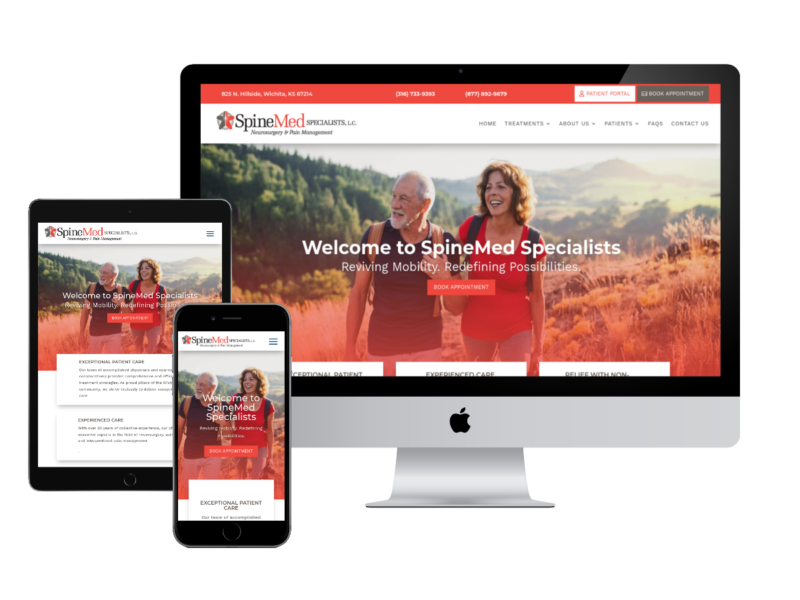The image showcases a cohesive display of three electronic devices—a monitor, a tablet, and a cell phone—all presenting the same website. In the center of the setup is a monitor with a sleek black top edge and a distinctive silver outline at the bottom. The base of the monitor is also silver, adorned with the iconic Apple logo.

The website on display belongs to "Spine Med Specialists, LC," featuring a warm welcome message: "Reviving Mobility, Redefining Possibilities." At the heart of the website is a captivating image of two individuals—a senior man and a middle-aged woman—walking together, symbolizing restored mobility and vitality. A red banner with white text reading "Book Appointment" adds a call-to-action element to the site.

To the side of the monitor sits a black-bordered tablet, also displaying the same website. However, the tablet's screen reveals additional content, including two rectangular panels at the bottom, though the words within these panels are not discernible.

In the foreground, partially in front of the tablet, lies a cell phone. The smartphone screen mirrors the identical website content shown on both the monitor and the tablet, maintaining the same visual consistency and professional appeal across all devices.